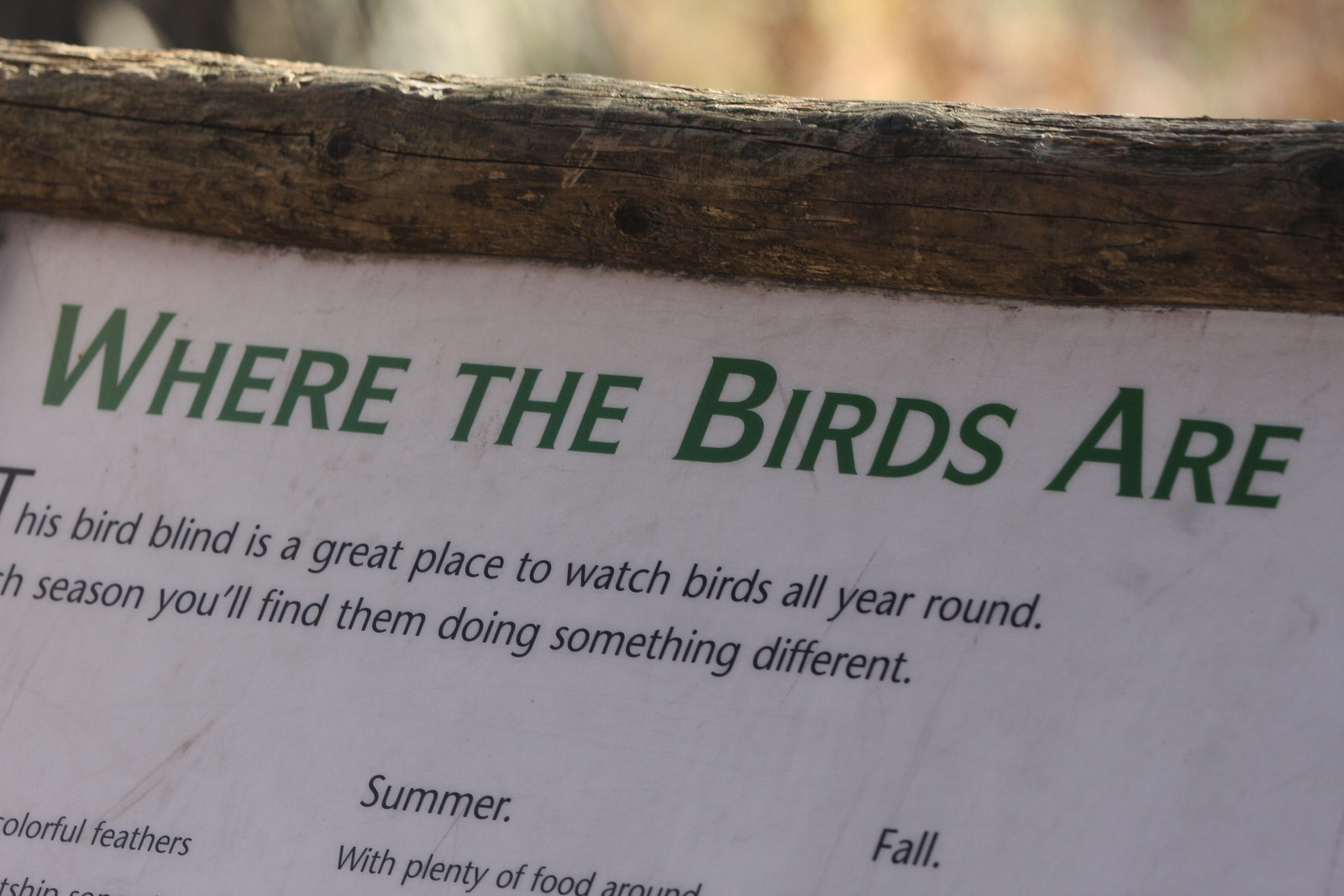This image features a close-up of an outdoor sign, embedded between two rough, untreated wooden posts at the top, reminiscent of tree branches. The sign itself appears to be a white plaque with a green, all-caps title stating "WHERE THE BIRDS ARE." Below the title, in smaller black letters, the sign reads, "This bird blind is a great place to watch birds all year round. Each season you'll find them doing something different." The sentences seem partially cut off, but there are mentions of "summer" and "fall," suggesting it details bird behaviors across different seasons. The background is blurry, hinting at a shaded outdoor environment with forest and some lighted grass visible.